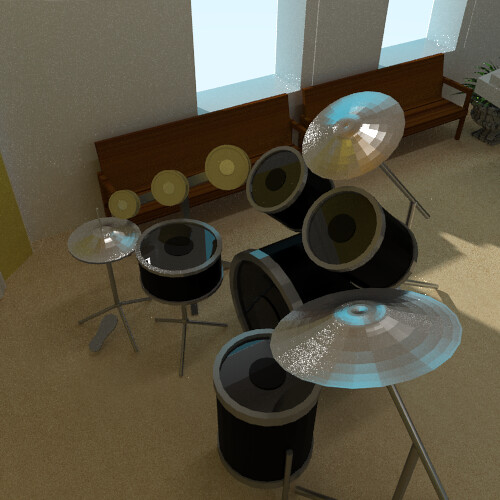The image depicts an indoor setting featuring a 3D modeled or possibly computer-drawn drum set. The drum set comprises black, circular drums with silver edges and lighter gray sides. One of the drums has a foot pedal on the floor. The setup includes a metallic circular cymbal, which is silver, and symbols above the drum set that are gold and silver.

The backdrop showcases an off-white wall adorned with two square glass windows without any design. In front of the windows, there are two reddish-brown wooden benches placed side by side. Additionally, there is a potted plant with a stone-like pot situated to the right of the benches.

The flooring in the room is a light yellowish-brown color, providing a subtle contrast to the darker-colored drums and wooden benches. The entire image is presented in a rectangular format.